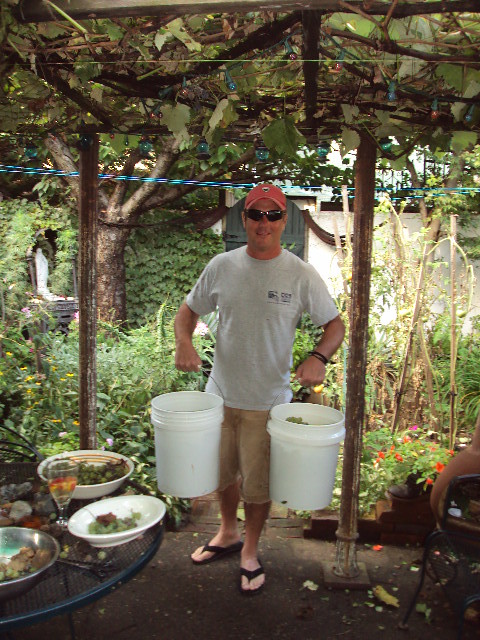In this image, a Caucasian man in his late 40s stands as the central figure, holding two five-gallon white buckets, possibly containing items from his garden. He is dressed casually in a gray, short-sleeved t-shirt, khaki shorts with frayed edges, a bright orange baseball cap, and black sunglasses, despite the overcast daylight. On his feet, he wears flip-flops. His wrist is adorned with a bracelet.

The setting is an intricately cultivated garden area. Behind the man, a walkway divides the garden, which features a variety of lush green plants, some trained with poles and others grouped together, hinting at meticulous care. Above, a wooden framework supports vines creating a sheltered area. Strung lights add to the charm of the garden space.

In the bottom left corner of the scene, an outdoor iron-style table with a wire mesh top is visible. The table is set with bowls containing an assortment of food, including fruits, salads, and possibly meat, along with a glass of water, suggesting a recent or upcoming meal. The overall atmosphere is serene and green, encapsulating the essence of a well-tended garden enclave.